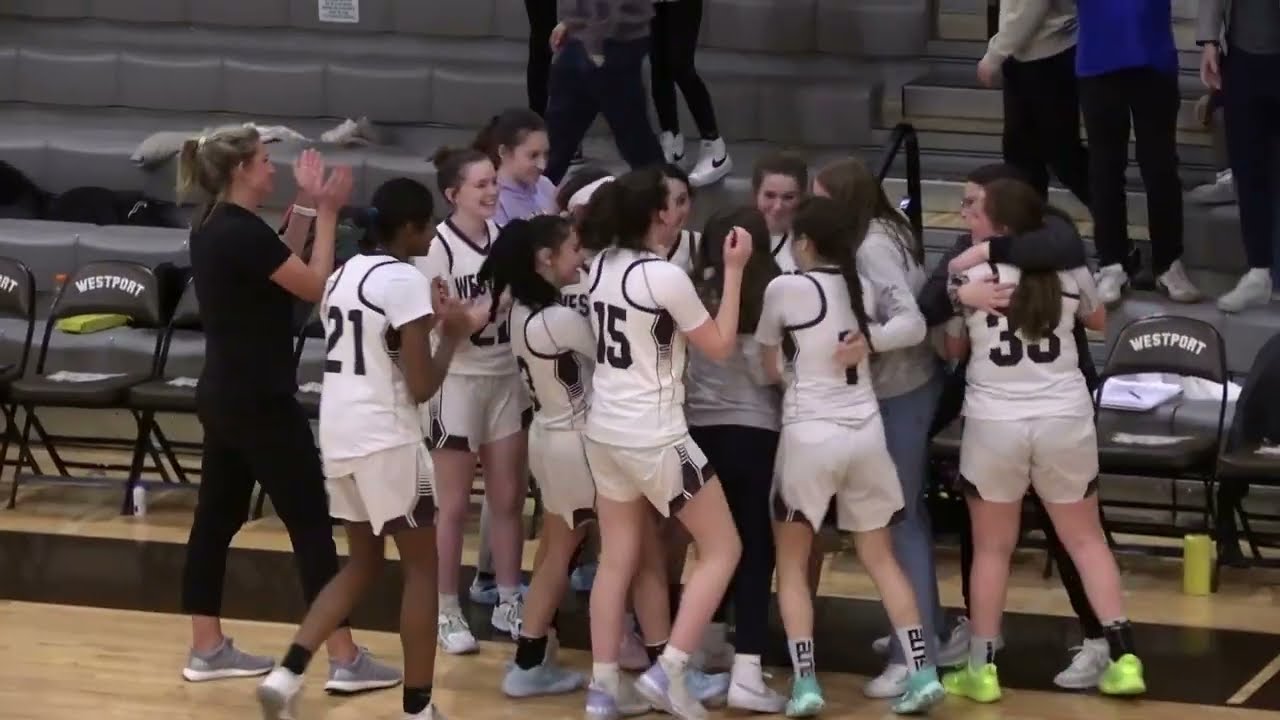This image captures a celebratory moment of a girls' high school basketball team from Westport. Approximately 10-12 young athletes, of mixed races, are gathered in a joyous huddle on a light brown wooden gymnasium floor, marked by dark horizontal lines. They are all dressed in white jerseys and shorts, adorned with black numbers on their backs, such as 15, 21, and 35. Their feet are clad in various colored sneakers, including gray, purple, green, and blue. 

In the midst of the group, a girl with the number 15 on her back stands out. The girls are visibly happy, likely celebrating a victory, evident from their embraces and smiles. Standing beside them is the coach, a woman with blonde hair who is clapping, dressed in a black short-sleeved shirt and black capri leggings. 

The background shows black folding chairs with "Westport" printed in white, some spectators in gray bleachers, and black railings with steps. The crowd appears to be either cheering or preparing to leave, contributing to the lively atmosphere of the scene.